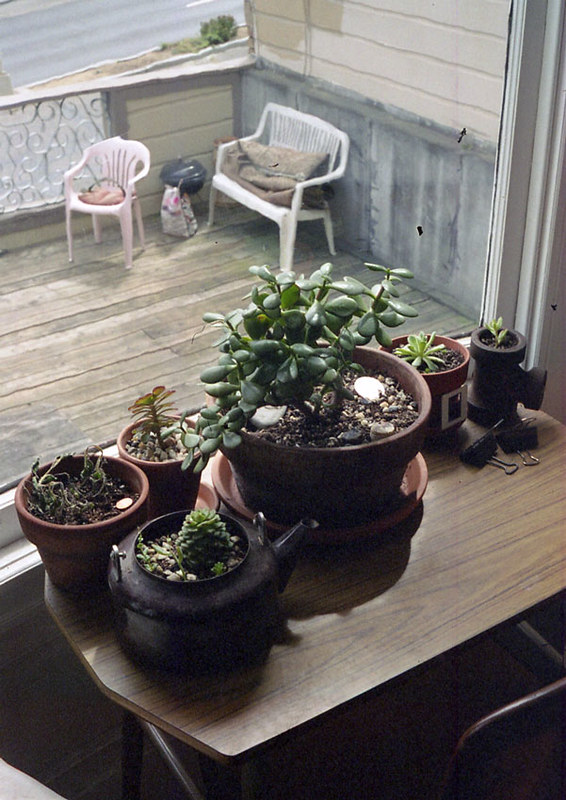The photograph captures an indoor scene with a wooden, brown-laminated table serving as the focal point. On this table, there are six distinct flower pots, each containing various plants. The central pot is larger and features a vibrant green plant, while the surrounding pots hold a mix of succulents, a tiny tree, and sprouting plants. One of the pots is shaped like a teapot, adding a whimsical touch. Notably, some plants appear healthier than others, with one seemingly dying.

In front of the table is a plastic chair. The backdrop of this indoor scene includes a large picture window framed in white, providing a clear view of an outdoor deck area. The weathered, light-stained wooden deck features two plastic chairs, one white and one pink, each draped with a blanket. Beside the chairs, there is a small charcoal grill with a bag of charcoal nearby. Beyond the deck's elaborate white patterned railing, the view extends to a street separated by a strip of grass and bushes, adding depth to the overall scene.